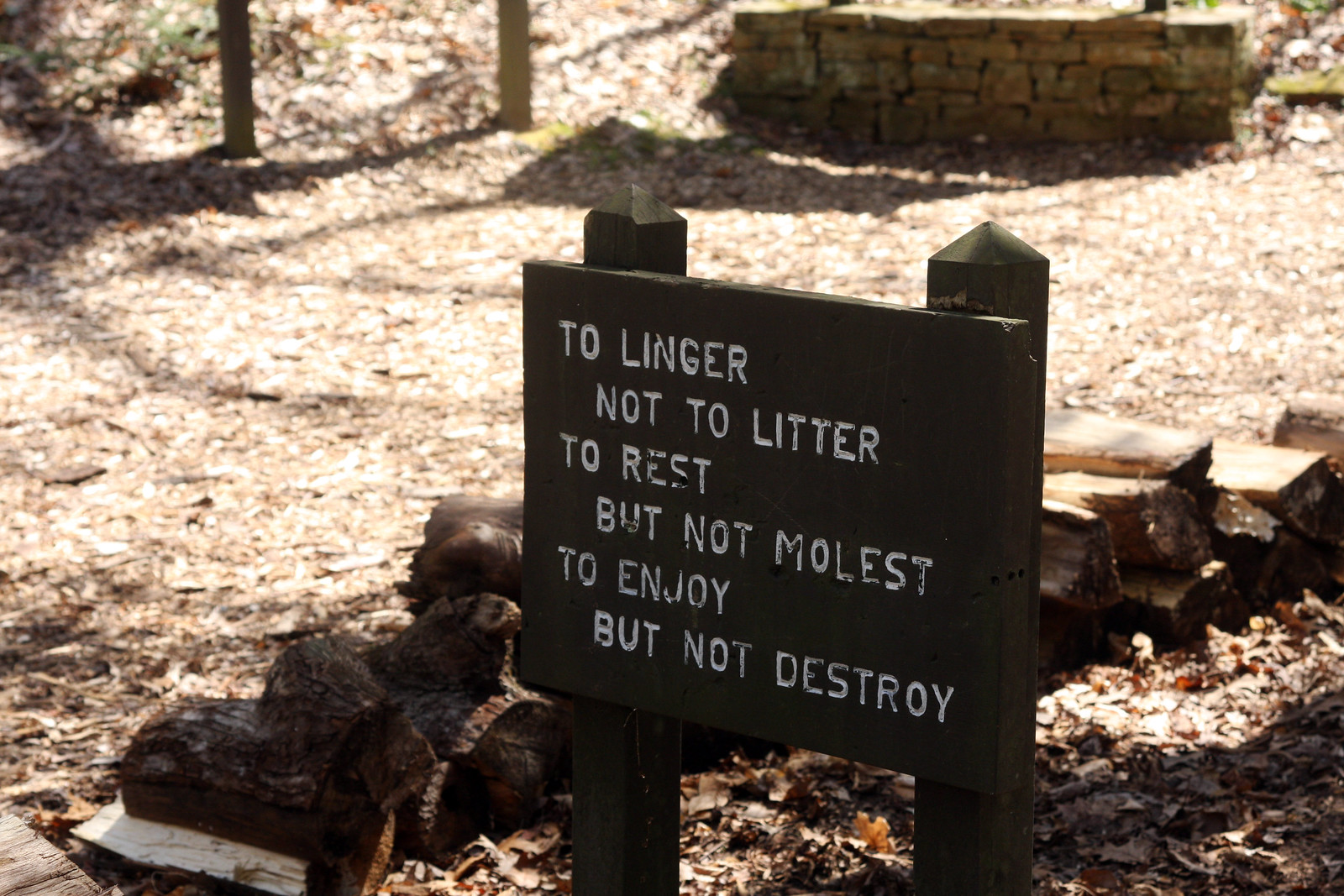The image showcases a small, brown, wooden sign positioned centrally amidst an outdoor setting. The sign, elevated on two wooden posts, features an emphatic message carved into it and painted in white: "To linger, not to litter. To rest, but not molest. To enjoy, but not destroy." This sets a tone of respectful usage for the area, suggesting it is a rest site or camping area.

Behind the sign, rows of neatly stacked cut logs are visible, likely for firewood use. The ground is carpeted with a thick layer of brown leaves, hinting at a natural, forested environment. Sunlight filters through, illuminating a pathway with scattered wood chips and dead leaves, adding to the serene ambiance. In the background, a small stone wall constructed of field stones is visible at the top right, while two wooden bars and possibly another sign can be seen towards the top left. Tree shadows dance on the pathway, enhancing the sense of tranquility in this rustic outdoor scene.